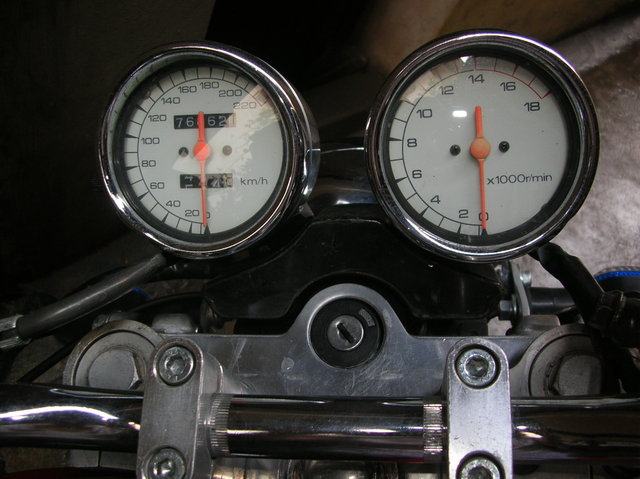This detailed photograph captures a sophisticated metal contraption prominently featuring two gauges, set against a textured, gray fabric backdrop that transitions from shadow on the left to light on the right. The fabric background is out of focus, emphasizing the sharp detail of the mechanical foreground.

The contraption itself is constructed from shiny metal components, including a horizontal bar with rounded ends and a central black component featuring a keyhole-like design with an empty slit. Directly in front of this bar, running along the bottom of the frame, is another horizontal metal rod adorned with metallic clasps, also gleaming in the light.

Atop this metal assembly sit two gauges, both encased in shiny metal rims with glass fronts. Each gauge has a semicircular scale ranging from the bottom to the upper right, reaching approximately the 1 o'clock position. 

The left gauge's scale ranges from 0 to 220, with an orange needle indicating 0. Within this gauge, a smaller, black-and-white odometer-like display reads 76,000, followed by an obscured digit, and then 62. Beneath this, another partially visible number labeled "kilometers per hour" can be discerned.

The right gauge mirrors the left in design but with a different scale, running from 0 to 18 in increments of 2. An orange needle also points to 0. This gauge is labeled "times 1,000 R per minute."

The meticulous construction and detailing of the mechanisms are clearly highlighted, showcasing the complexity and precision of the apparatus.